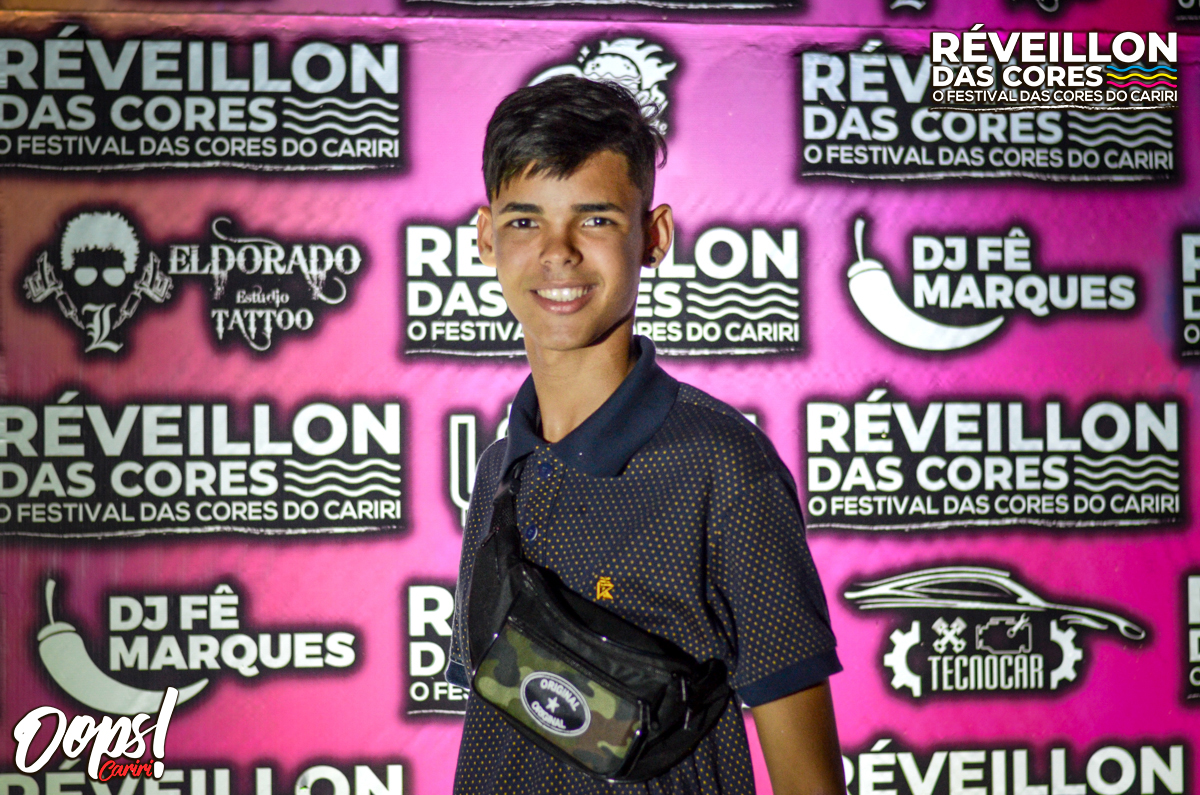This photograph, taken indoors, features a young man, either white or Hispanic, likely in his late teens. He has light brown skin and short black hair, shaved on the sides. He is dressed in a gray polo shirt adorned with orange polka dots and is smiling at the camera in a three-quarter stance. A camouflage cross-body bag, worn across his chest, prominently displays a black oval logo with the word "Original" written on it, and the lower left-hand corner of the bag reads "OOPS!" with an exclamation point. 

The backdrop consists of a vibrant purple sign with various white logos and text. Dominating the signage are the words "REVEILLON DOS COROS" and "Festival dos Coros do Caribe, Tecno Car," written multiple times across the background, including in the top-right corner. Additional text hints at other festival sponsors and DJs, adding to the festive atmosphere. The image captures not only the youthful, joyous essence of the subject but also the lively, celebratory mood of the event he is attending.